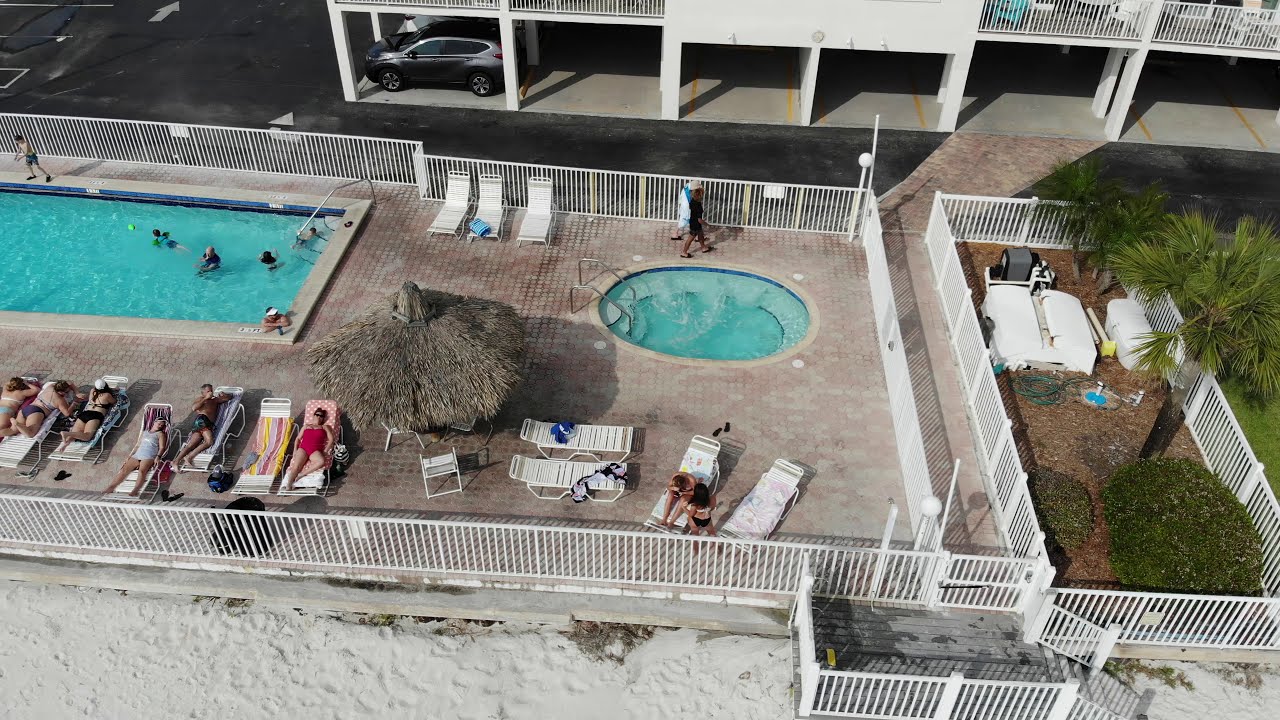The aerial photograph captures a lively motel pool scene with great detail. At the bottom left of the image, a poolside area showcases people lounging on chairs and basking in the sun, bordered by a white fence. Adjacent to them lies a rectangular swimming pool with a silver handrail and steps, where several guests are seen swimming and one individual stands beside it in the upper left corner. Centrally located is a circular pool with steps flanked by silver handles, adding to the aquatic charm. Beyond this, two individuals are seen walking towards the right. A parking lot is visible above the fenced barrier, where a silver car is parked in one corner. On the right side, a palm tree is enclosed by another white barrier, contributing to the tropical ambiance. In the bottom right corner, barriers indicate the presence of a gate, providing access to this inviting pool area. Overall, the photograph, taken from about 20 to 30 feet above, offers a comprehensive view of the pool's layout and the serene environment, with the concrete platform and surrounding white sand enhancing the scene's appeal.